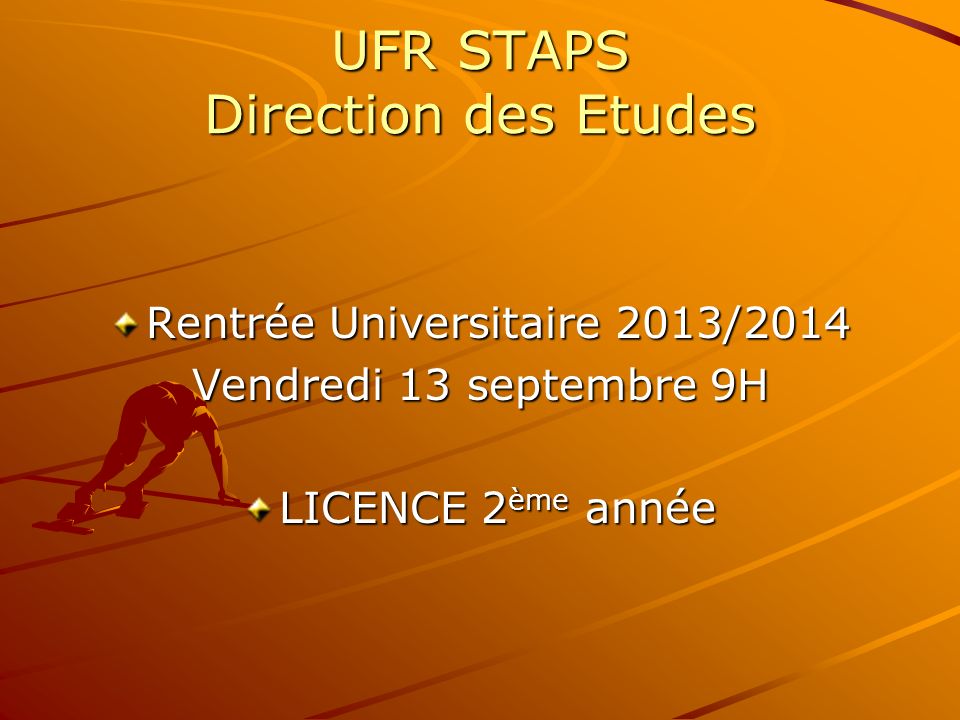The image features a vibrant, bright orange background with a detailed outline of a track, illustrated by several lines forming oval shapes. Positioned in the lower left quadrant is a silhouette of a track star crouched in a starting position, hands resting on the track. Across the top of the image, in a bold yellow font, the text reads "UFR STAPS Dirección de Études." Below this, two golden bullet points provide additional event information: the first states, "Rentrée Universitaire 2013-2014 Vendredi 13 Septembre 9H," and the second reads, "Licence 2MA Année." The overall color scheme includes orange, yellow, black, white, red, and maroon, and the layout suggests it is an advertisement for an upcoming university event related to track and field.